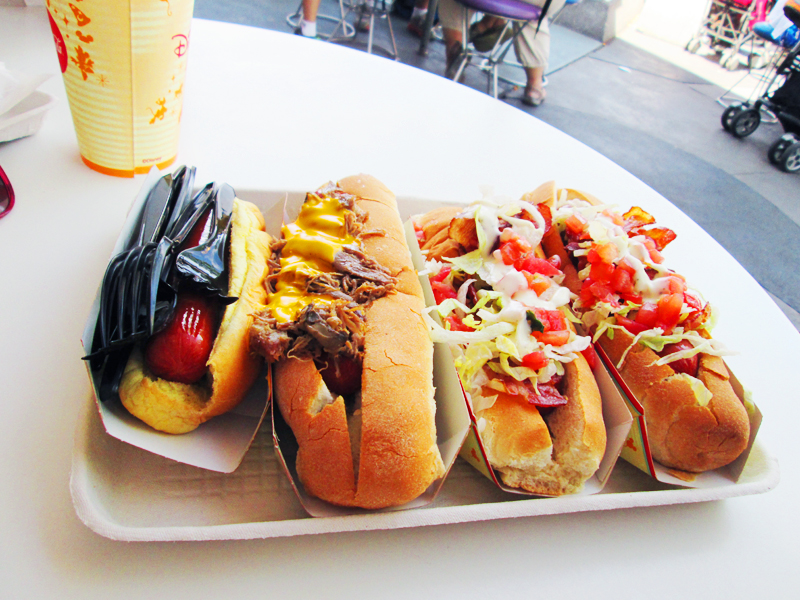In this detailed close-up photograph, we are looking at a white round table, likely in an outdoor dining area at Disneyland as suggested by the yellow paper cup featuring Disney characters and a prominent "D" logo. On the table, there is a cardboard tray holding four hot dogs, each in its own little holder. The leftmost hot dog is plain and topped with at least three or four plastic forks. To the right of that is a hot dog covered in what appears to be shredded meat and yellow cheese, housed in an oversized bun with a noticeable brown crust. The next hot dog features a lightly toasted bun piled with coleslaw, and possibly bacon. The rightmost hot dog mirrors the third, but also has visible tomato slices alongside coleslaw and bacon. The background reveals a gray concrete ground, a purple seat with silver legs, a stroller with black wheels, and glimpses of people’s feet, enhancing the bustling, casual atmosphere of the setting. It appears to be daytime, and the image has a slight retro vintage aesthetic.